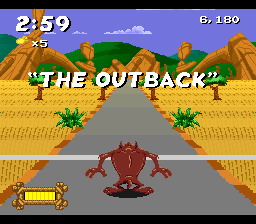This is a detailed screenshot from a Tasmanian Devil video game. The image shows the Tasmanian Devil from Looney Tunes standing with his back to the viewer on a dark gray road, slightly spreading his legs and positioning his arms at his sides with his hands pointing down. His fur is a dark chocolate brown, and he sports a tail and pointed ears. Behind him, there is a circular shadow.

On the left side of the screen, a small HUD displays a series of gold crosses and a bar filled with gold rectangles separated by red lines. A light gray line runs horizontally across the road, denoting the start line. Along both sides of the road are soil sections that transition from dark chocolate brown to lighter brown, forming a pattern that extends into the distance. The golden soil sections are streaked with dark chocolate brown lines, resembling rolling hills.

The scene features several trees with dark chocolate brown trunks, light green leaves, and darker green edges. There are also dark green pointy plants with lighter green accents. In the background, light brown mountains with dark brown highlights and forest green mountains create a 3D effect. The sky above is a purplish-blue with white clouds tinged with purple, greenish-blue, or bluish-gray hues.

At the top of the screen, a timer reads 2:59 in white, accompanied by an icon that shows "X5" in gold. On the upper right, a score of 6,180 is displayed in white. In the center of the screen, the text "THE OUTBACK" appears in bold, all-caps white letters within quotation marks, signifying the game's section.